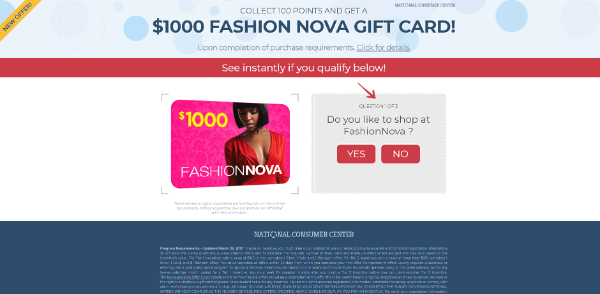This webpage features an alluring offer for a gift card, presented in a visually dynamic layout characterized by bold and contrasting colors. Dominated by hues of blue and red, with white and black fonts for textual content, the page immediately draws the viewer's attention to its central elements. 

At the top, a light blue pill bar adorned with floating blue bubbles contains an enticing call-to-action: "Collect 100 points and get a $1,000 Fashion Nova gift card upon completion of purchase requirements. Click for details." Beneath this, a prominent red bar invites users to "See instantly if you qualify below."

The main focal point of the page is a vivid image of the gift card, positioned to the left center. The gift card boasts a hot pink background and prominently features an elegant African-American woman with blunt-cut black hair, wearing a red V-neck dress. In bright yellow font, the card declares its value as $1,000, with the Fashion Nova logo displayed at the bottom.

To the right of the gift card image, a gray box poses the question, "Do you like to shop at Fashion Nova?" Accompanied by a red arrow pointing to it, this box further features pill-shaped buttons in red, labeled "Yes" and "No," which users can click to respond.

Completing the page, the bottom section includes a navy blue bar with "National Consumer Center" written at the top in white font. A tiny white disclaimer text follows at the very bottom, ensuring all legalities are covered. 

The entire composition of the webpage is designed to captivate interest, provide clear instructions, and drive engagement through its colorful, strategically arranged elements.